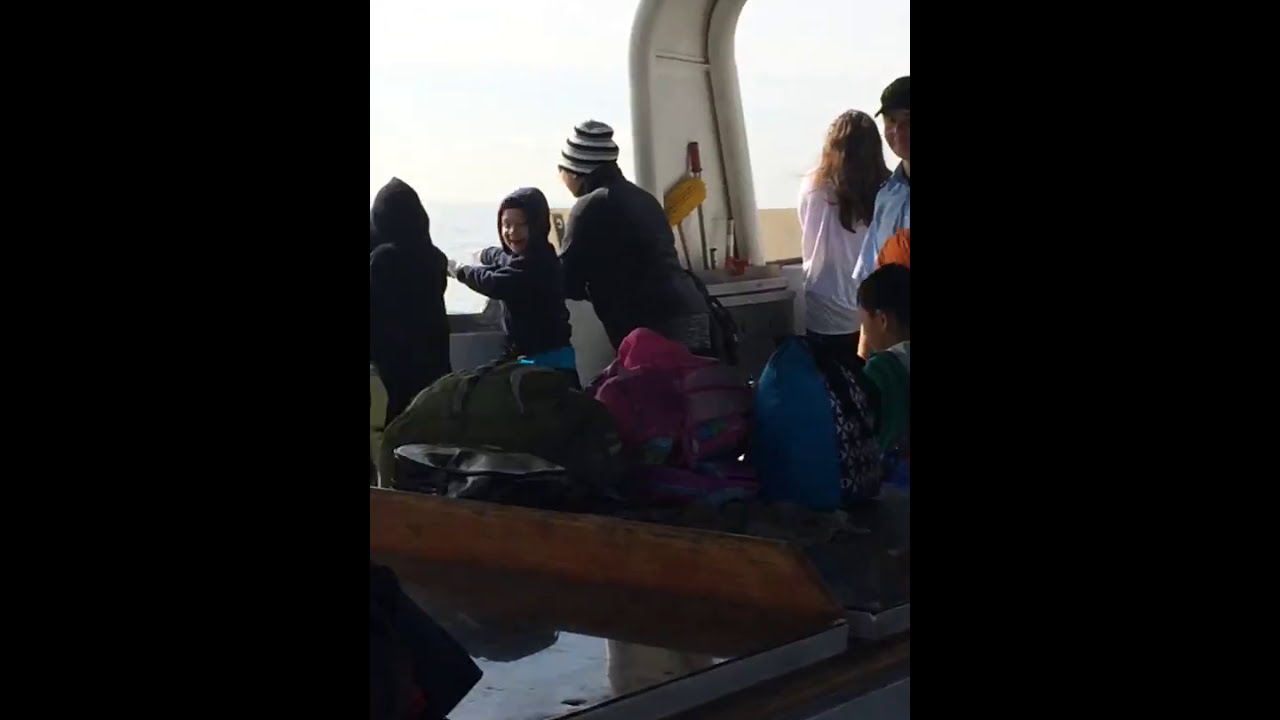In this photo, framed with black vertical bands on the left and right sides, we see a group of six people—three children and three adults—inside what appears to be the interior of a ferry or boat. The setting suggests a chilly day, as everyone is dressed in jackets and beanie hats. The focal point is a shiny brown table at the bottom of the image, cluttered with large, bulky bags in green, reddish, and blue hues. 

To the left, two little boys in black hoodies catch the eye; the second boy from the left looks back at the camera, smiling warmly and pointing forward, his brown skin glowing with joy. Beside these children stands a man in a long-sleeved black coat and a hat with gray, white, and black horizontal stripes. Further to the right, a supportive beam extends upward, adding to the structural detail of the space. 

On the right side of the beam, two more adults—one female and one male—are accompanied by another child, focusing their attention outside. Through the windows, the pale blue sky with streaks of white clouds and a faint hint of grayish water below create a serene backdrop. The overall scene suggests a sense of travel and togetherness, framed against the subtle beauty of a cold, yet calm, outdoor setting.